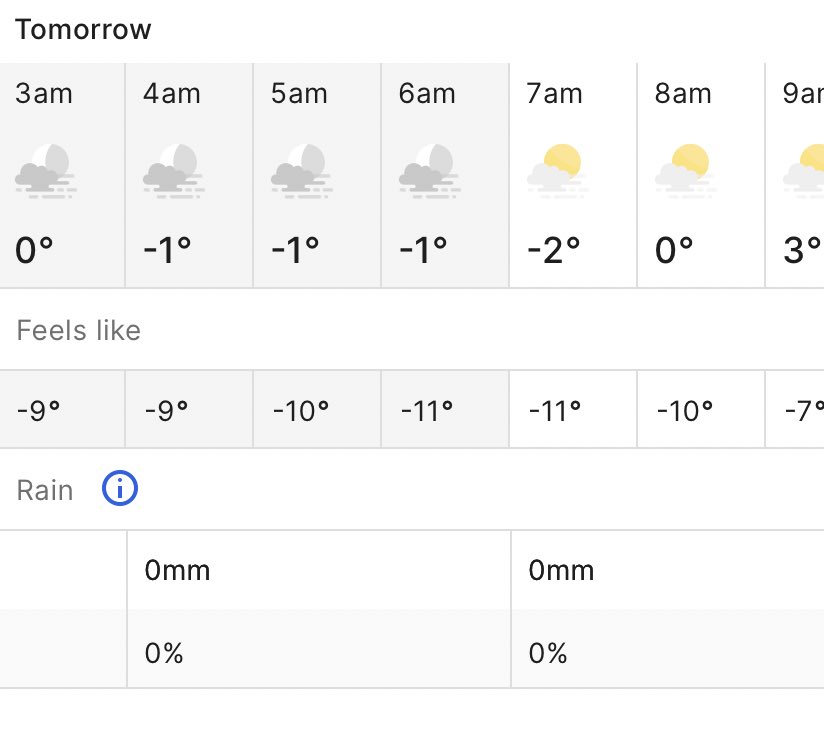A detailed screenshot from a weather app displayed against a clean white background, organized into several horizontal rows. At the top of the screen, the forecast for "Tomorrow" is shown, followed by hourly time slots: 3 AM, 4 AM, 5 AM, 6 AM, 7 AM, 8 AM, and 9 AM. Each time slot features an icon indicating weather conditions. From 3 AM to 6 AM, the icons show the moon behind a cloud, signifying partly cloudy nighttime conditions. From 7 AM to 9 AM, the icons depict the sun behind a cloud, designating partly cloudy daytime conditions.

The temperature readings for these hours are displayed beneath each time slot: 0°C at 3 AM, -1°C at 4 AM, -1°C at 5 AM, -1°C at 6 AM, -2°C at 7 AM, 0°C at 8 AM, and 3°C at 9 AM. Below the temperature readings are the "Feels like" temperatures: -9°C at 3 AM, -9°C at 4 AM, -10°C at 5 AM, -11°C at 6 AM, -11°C at 7 AM, -10°C at 8 AM, and -7°C at 9 AM.

Additionally, there is a section labeled "Rain" accompanied by a blue circle icon featuring an eye, intended for more information. This section indicates that there is 0 millimeters of rainfall and a 0% chance of precipitation throughout these hours.